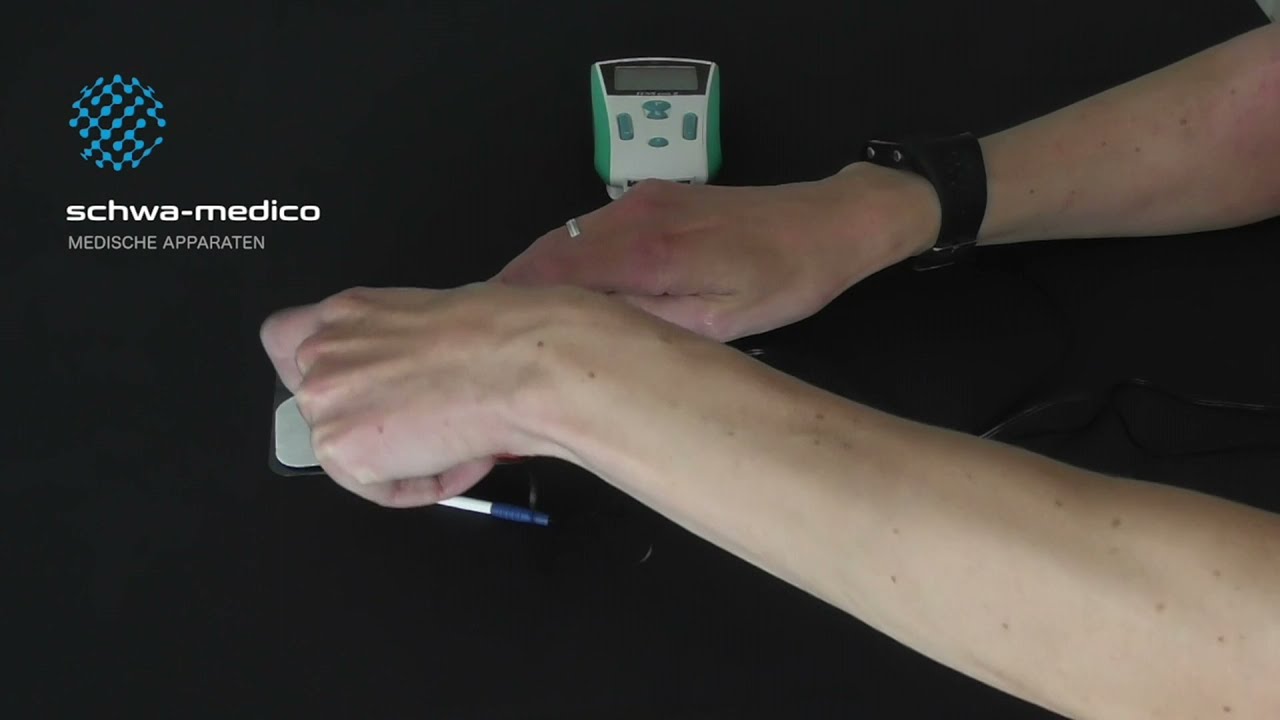The image depicts a scene that looks like a screengrab from an informational or instructional video, featuring a black background and two hands that appear to be working with a medical device. The person's right hand, adorned with a black watch and a silver ring on the middle finger, grasps a grayish-white pad with a small blue piece attached to it. The left hand is folded into a fist and also holds part of the device. Behind the hands is a green and white panel with an LED screen. In the top left corner of the image, a checkered blue and black circular logo is visible, with the text "Schwa-Medico" and "MEDISCHE-APPARATEN" written underneath. This setup suggests the image is about demonstrating or explaining the use of this piece of medical equipment.